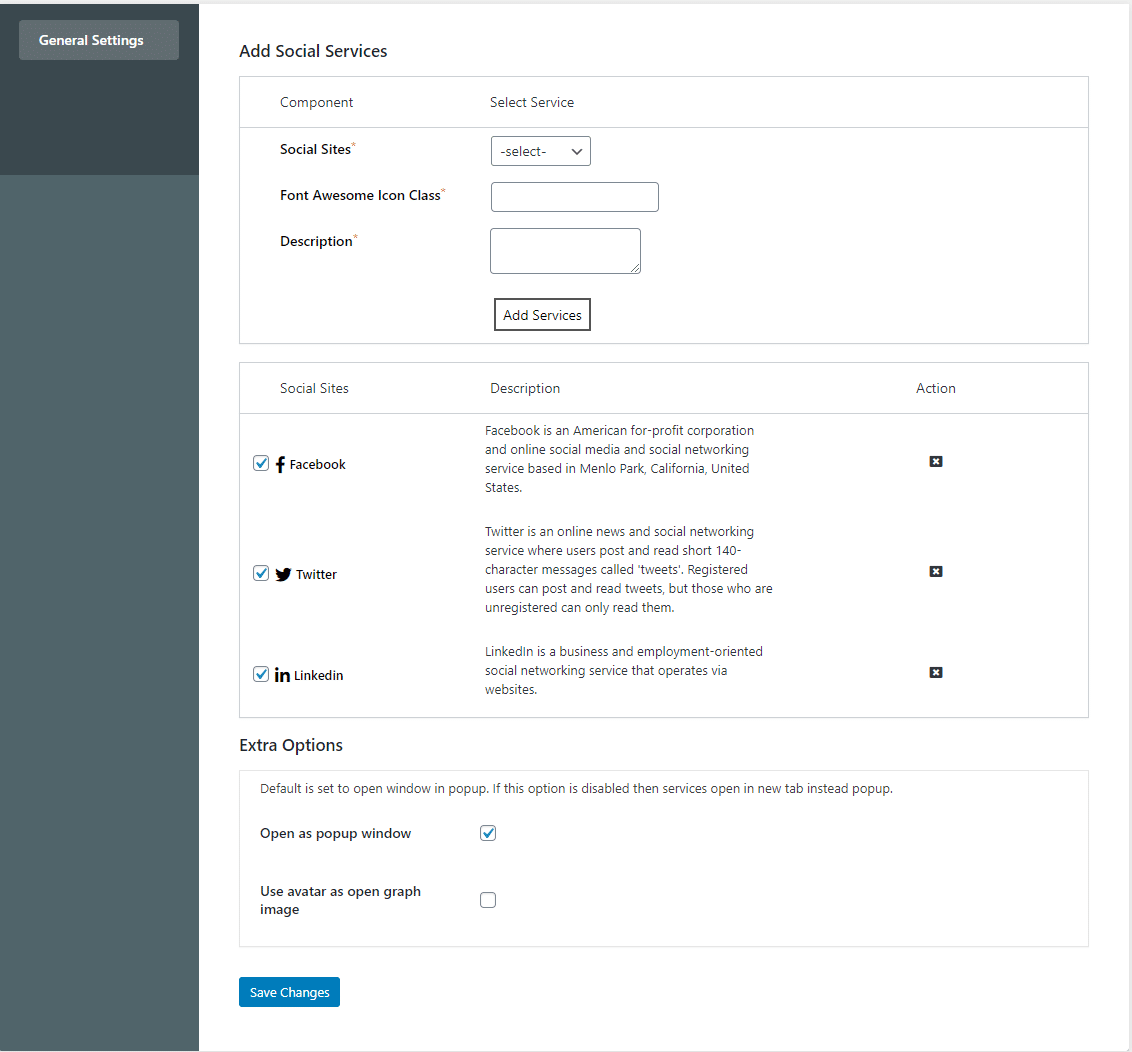The image displays a user interface for configuring social media settings within a web application. At the top of the main section, the heading reads "General Settings" in white text on a grey background. The UI is divided into two main sections: a dark grey and black sidebar menu on the left, and a white main form area on the right.

In the main form area, the top section is labeled "Additional Social Service." Below this heading, there are various input fields and options:
1. A dropdown menu labeled "Component."
2. A dropdown menu labeled "Select Service."
3. Another dropdown labeled "Social Site."
4. An input field for "Font."
5. An input field for "Icon Class," currently empty.
6. A text area for "Description," also empty.

At the bottom of this section, there is a button labeled "Add Services."

The form continues with sections detailing different social sites. Each site has:
- A "Social Site" label.
- A corresponding description.
- An action button represented by a black cross or 'X.'

To the right, a list of social sites, each with a blue checkmark indicating they are selected, includes:

1. **Facebook**
   - Description: "Facebook is an American for-profit corporation and online social media and social networking service based in Menlo Park, California, United States."
2. **Twitter**
   - Description: "Twitter is an online news and social networking service where users post and read short, hard and pointy character messages called tweets. Registered users can post and read tweets, but those who are unregistered can only read them."
3. **LinkedIn**
   - Description: "LinkedIn is a business and employee-oriented social networking service that operates via website."

At the bottom of the form, the "Extra Options" section includes:
- A checkbox for "Open window in a pop-up." If this option is disabled, the window will open in the top instead of pop-ups.
- A selected option for "Open as pop-up."
- An unselected option for "Use avatar as Open Graph image."

Finally, at the bottom, there is a blue button labeled "Save Changes."

This detailed configuration form allows users to manage various aspects of social media integration within the application.